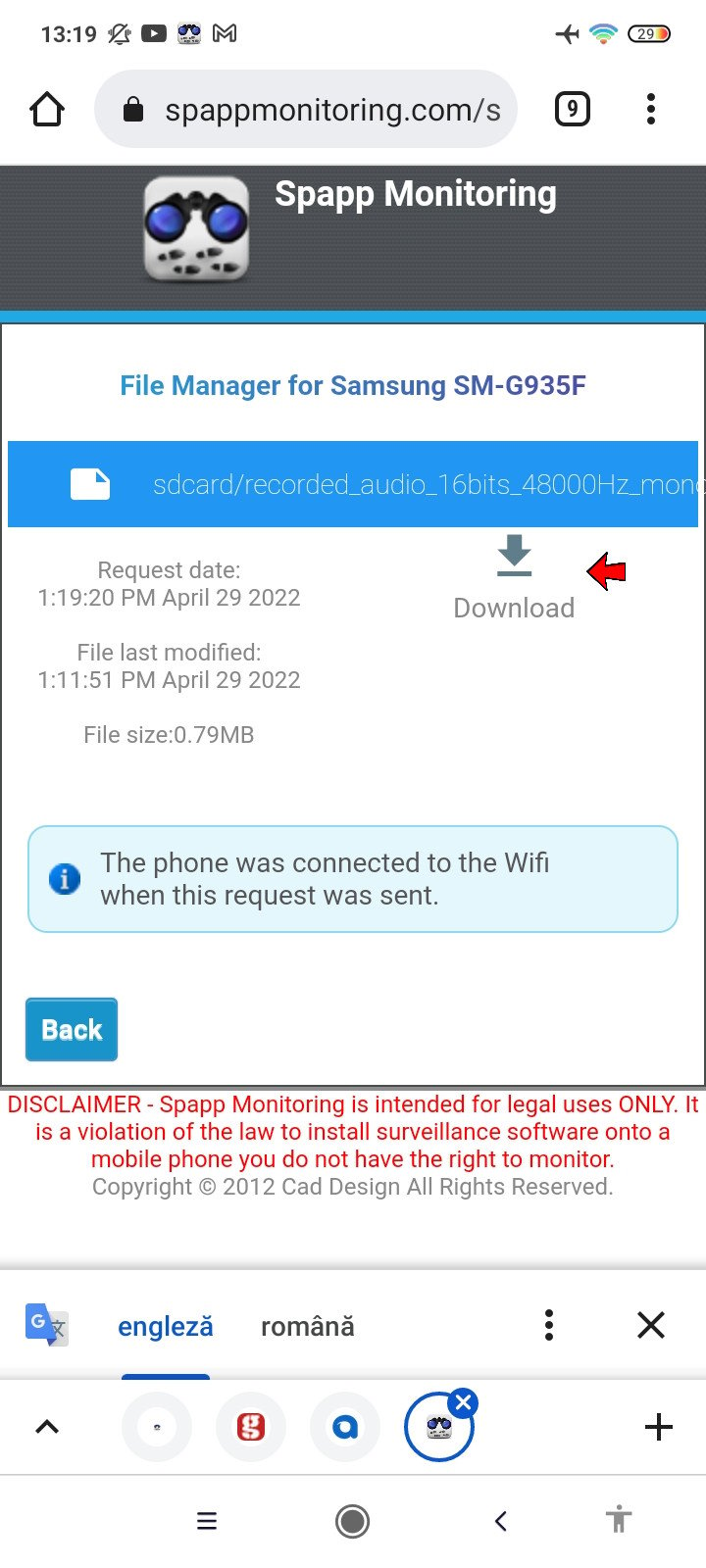The image depicts a smartphone screen in Airplane Mode, with colorful icons and notifications visible at the very top. The Wi-Fi signal icon is rainbow-colored, and the battery level is at 29%. 

At the top of the screen, there is a gray search bar displaying "SPAP monitoring.com." Next to it, a house icon signifies the home page, and a notifications icon shows the number nine. 

Below the search bar, a dark gray header reads "Snap Monitoring," featuring a logo of black and blue binoculars alongside four small footprint icons. It also mentions "File Manager for Samsung SM-G935F" followed by a lengthy file number. The request date and time are listed as "1:19:20 PM April 29, 2022."

Two arrows, one blue and one red, labeled "Download" are present. Additionally, a blue rectangular box explains that "The phone was connected to the Wi-Fi when this request was sent." A blue back button appears, along with various icons at the very bottom of the screen.